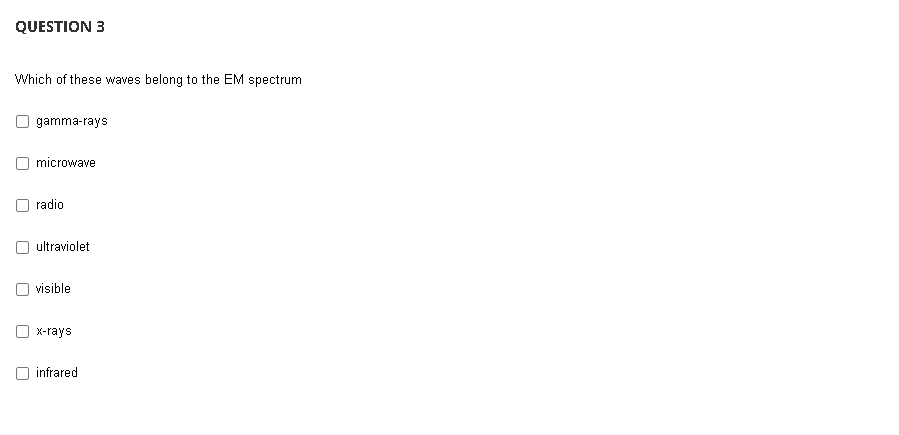This is a detailed caption of a screenshot depicting a science-related trivia question. The image presents a quiz interface with a black background and a prominently white box containing the query and response options. At the top of the white box, the text "Question 3" serves as a header. Below this heading, the question reads: "Which of these waves belong to the EM spectrum," notably missing a question mark. The available answers include "Gamma rays," "Microwave," "Radio," "Ultraviolet," "Visible," "X-rays," and "Infrared," each accompanied by a checkbox, allowing multiple selections. The image does not provide information on the correct answers nor does it indicate its source or the platform it is from. The design emphasizes a clean, straightforward quiz layout, although it leaves some ambiguity in appearance and context.